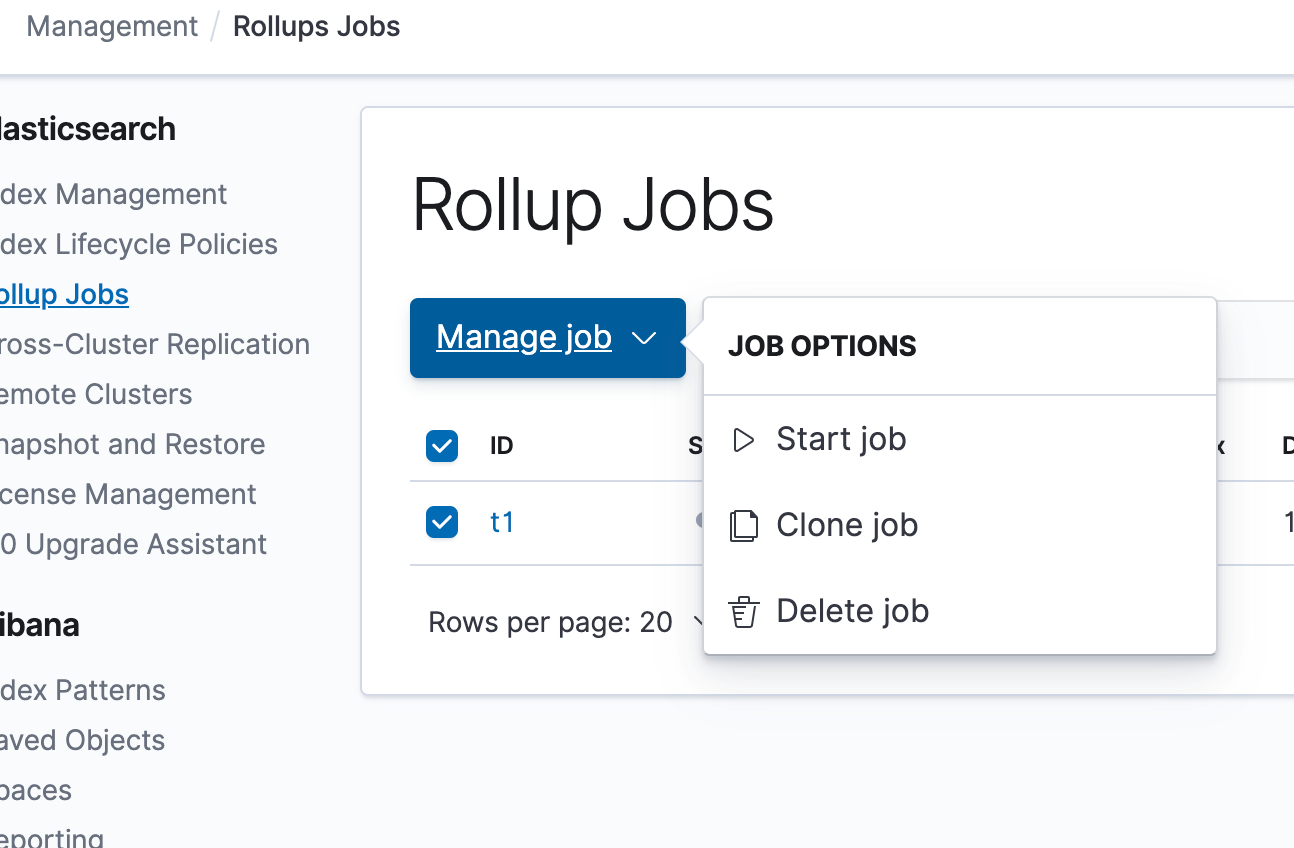The web page displayed is dedicated to the management of rollup jobs. On the left side, there is a section with truncated text that reads "Index Management," followed by options such as "Index Lifecycle Policies," "Rollup Jobs," "Cross-Cluster Replication," "Remote Clusters," "Snapshot and Restore," and “License Management.” Additional components listed include "Index Patterns," "Saved Objects," "Spaces," and "Reporting."

In the center of the page, a white box prominently displays "Rollup Jobs." There are blue tabs with a drop-down arrow labeled "Manage Jobs," providing options such as "Start Job," "Clone Job," and "Delete Job." Each job option is accompanied by an icon: a right-facing arrow next to "Start Job," a copy icon next to "Clone Job," and a trash can next to “Delete Job.”

Below these options, there are two lines for entries indicating job details, with checkboxes allowing selection. One entry checkbox is highlighted in blue, featuring the label "ID" next to a drop-down arrow. Due to an overlapping pop-up, the remaining part of this section is obscured.

At the bottom of the white box, there is a blue square with a white checkmark next to the label "Rows Per Page: 20" which also includes a drop-down arrow for adjusting the number of rows displayed.